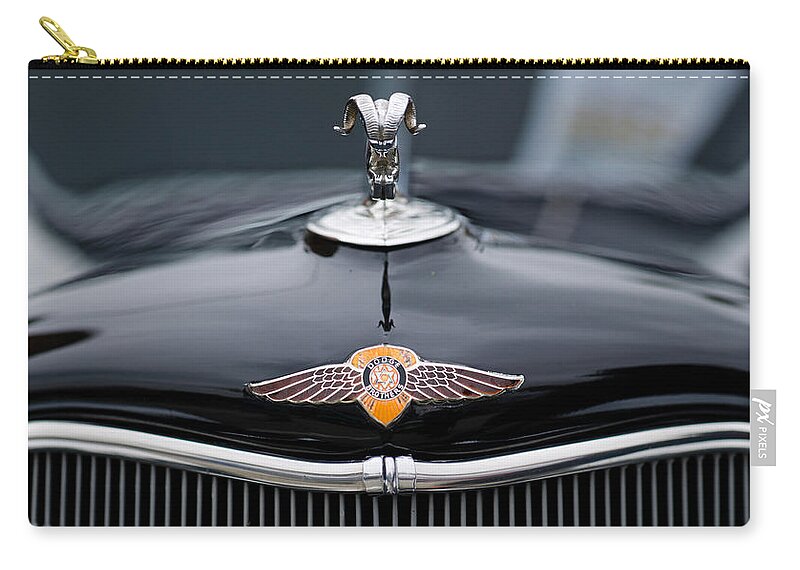This image features the front end of a glossy black Dodge vehicle, likely a pickup truck given the prominent Ram hood ornament. The Dodge emblem with orange and brown wings is centered on the sleek, silver grill, which curves up at both ends. Reflections in the glossy paint suggest the vehicle is in pristine condition. A gold zipper frames the top of what appears to be a case or bag in the background, hinting at it possibly being a pencil holder or makeup case. A small tag on the right-hand bottom corner reads "PX Pixels," adding a unique detail to the composition.